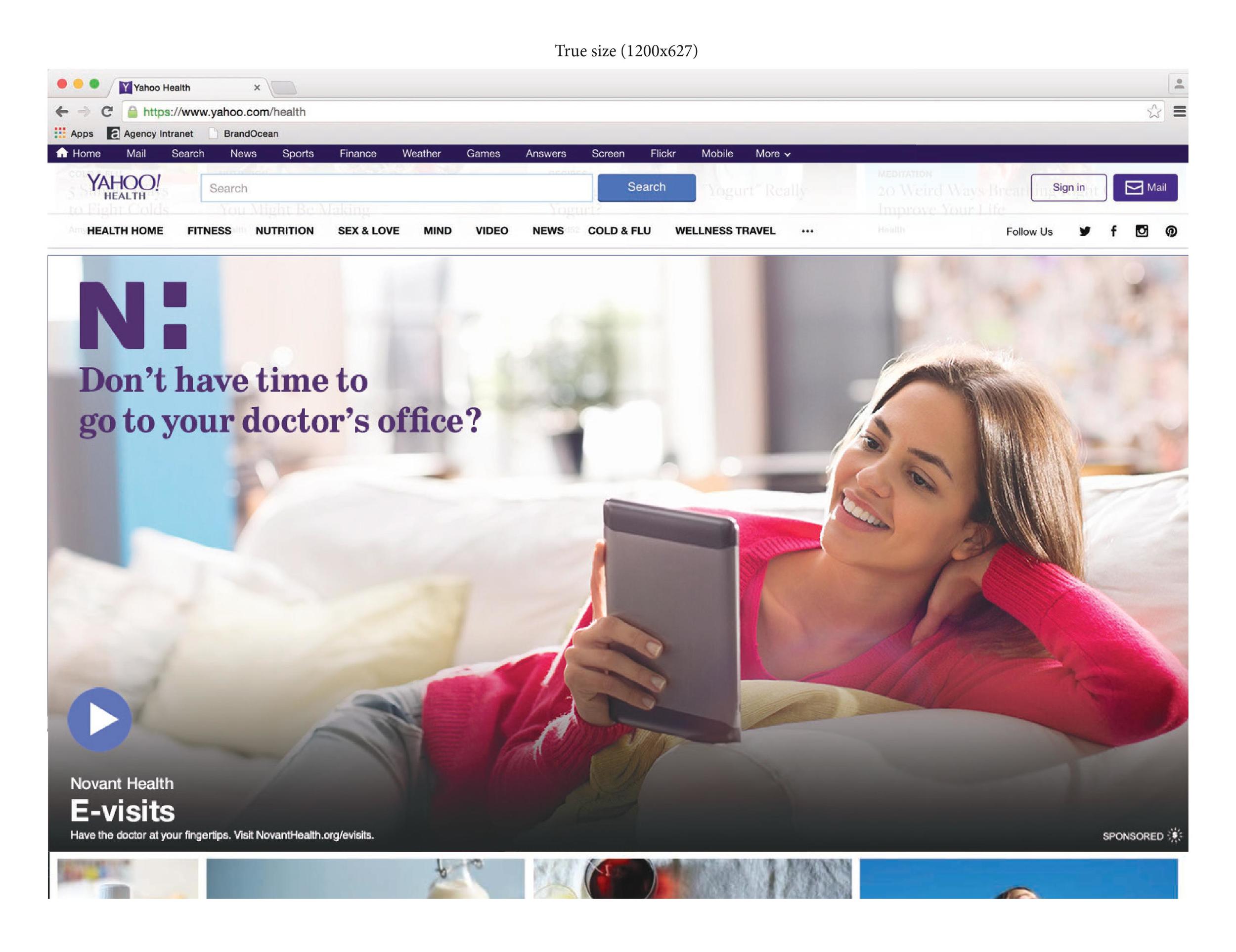**Caption:**

This screenshot captures the splash page for Yahoo Health at Yahoo.com. The webpage is designed with a clean and organized layout, beginning with a label at the very top specifying the true size of the image as 1200 by 627. The browser tab is appropriately labeled "Yahoo Health."

A purple navigation bar spans across the top of the page with tabs reading "Home," "Mail," "Search," "News," "Sports," "Finance," "Weather," "Games," "Answers," "Screen," "Flickr," "Mobile," and a "More" dropdown menu. Below this bar, the Yahoo Health logo is prominently displayed alongside a search bar, where users can type their queries.

To the far right, there is a sign-in section complete with a mailbox icon. Just below, there is a black navigational menu bar listing various health-related topics: "Health," "Home," "Fitness," "Nutrition," "Sex and Love," "Mind," "Video," "News," "Cold and Flu," and "Wellness Travel," followed by an icon to view more options. Next to these, icons encourage users to follow Yahoo Health on social media platforms including Twitter, Facebook, Instagram, and Pinterest.

The focal point of the image is a prominently displayed advertisement for Novant Health eVisits. The advertisement features a woman reclining on a couch, facing left. She is dressed in a red sweater and gray pants, holding a gray tablet in her right hand, while her left hand props up her head in a relaxed pose. She has shoulder-length brown hair and is smiling broadly, revealing her white teeth.

The text accompanying the image reads, "Don't have time to go to your doctor's office?" Below this, a blue button with a play arrow suggests the option to watch a video. Further text describes the service: "Novant Health eVisits – have the doctor at your fingertips. Visit NovantHealth.org/eVisits." The bottom right corner of the ad is marked with the word "Sponsored," indicating this content is a paid advertisement. 

Overall, the screenshot efficiently combines navigation and an attractive advertisement, poised to inform and engage users with its health-related content and services.